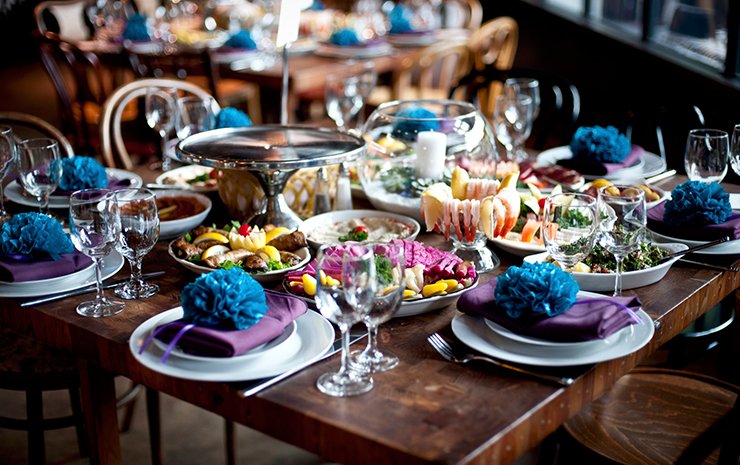In an indoor setting, the image captures a beautifully arranged dark wood table ready for what appears to be a special gathering, possibly a wedding party. The table, square in shape with dark wood chairs surrounding it, is meticulously set with an array of plates, most notably six plates with elegantly folded purple napkins, each adorned with a blue carnation-like flower. At the heart of the table lies a glass pedestal, empty but set to suggest it might hold a cake, and a centerpiece glass with a candle, surrounded by glasses filled with shrimp cocktail. Scattered around are various shallow white dishes containing different foods, including vegetables and meats, as well as empty wine glasses with stems and silverware placed next to the plates. In the upper right corner, a window provides a hint of natural light. The floor below is brown, either stained cement or tile. In the background, another table mirroring the same detailed place settings is visible, though slightly blurred, reinforcing the sense of a large, coordinated event. A door with glass panes is also discernible at the top right. The overall scene suggests a refined and ready-to-serve atmosphere, prepared for an intimate and elegant celebration.